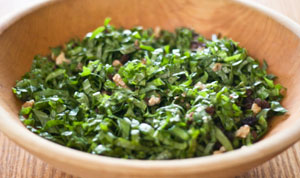This image is a close-up shot of a small wooden bowl placed on a light wooden table. The bowl contains what appears to be finely chopped and possibly muddled green herbs, most likely cilantro, intermixed with small golden flecks that could be seeds or a different kind of herb. This green garnish or mixture is the primary focus of the image. The detail and texture suggest it may be prepared for use as a seasoning or garnish, potentially for a marinade or to top a dish. Despite the low resolution, the freshness of the green herbs stands out vividly against the light brown wooden background.